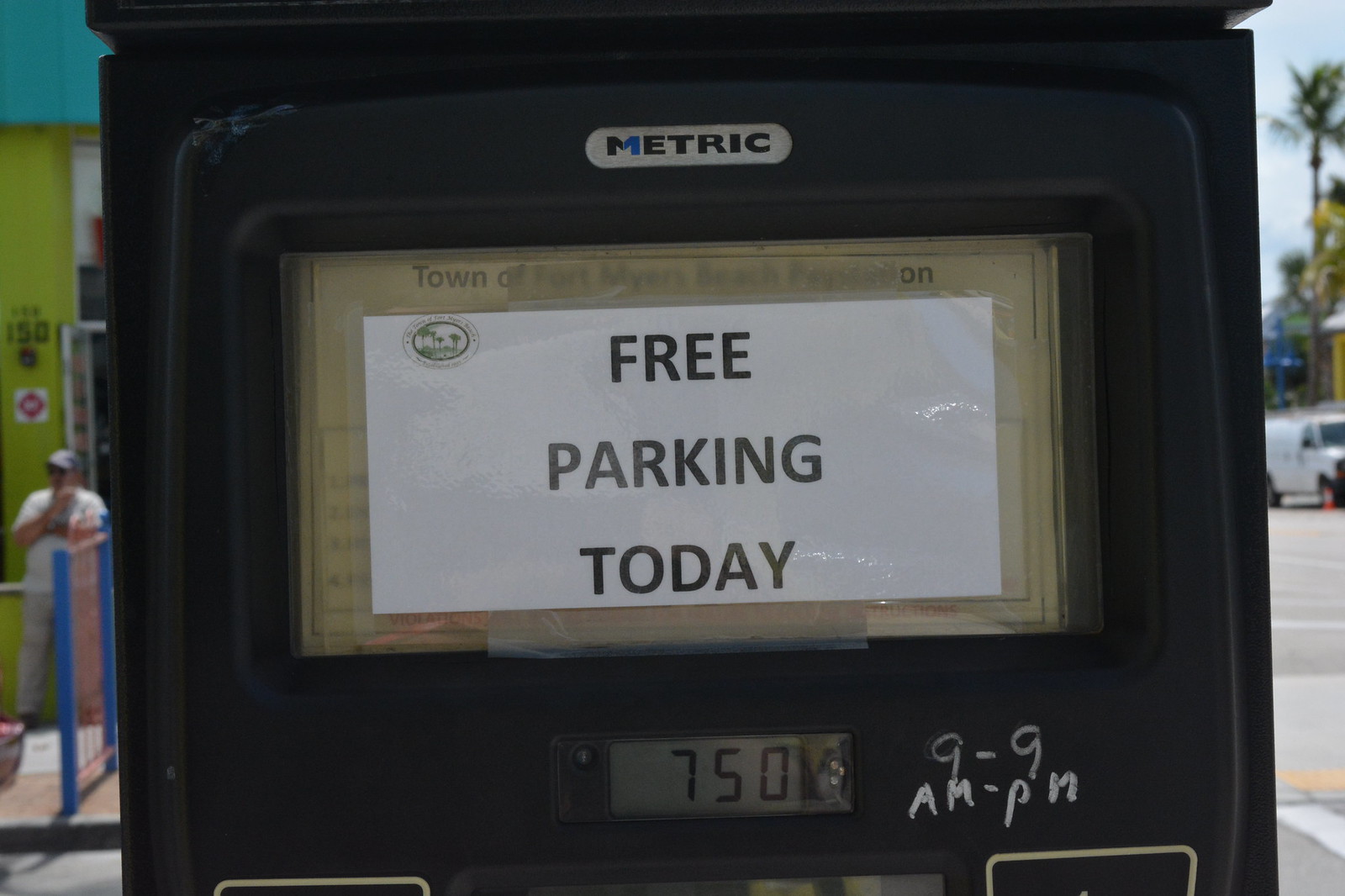This is a detailed picture of a parking meter affixed to the back of a black truck in a metropolitan area. At the top of the meter, there is a rounded rectangular label with the word "Metric" in black lettering on a white background. Below that, a white piece of paper taped to the meter’s screen displays the message "Free Parking Today" in black text, covering the usual digital display. Beneath this paper is a section that reads "750" in black on a gray background, resembling a timer or meter reading. Supplementing this, someone has written "9 to 9 a.m. to p.m." in white chalk on the lower right.

To the left of this setup, a man dressed in a white shirt is leaning against a green wall with a teal awning, separated from the truck by a blue fence or short black banister. In the background to the right, a white van is parked near a street, beside palm trees and a variety of buildings, with a vast blue sky overhead.